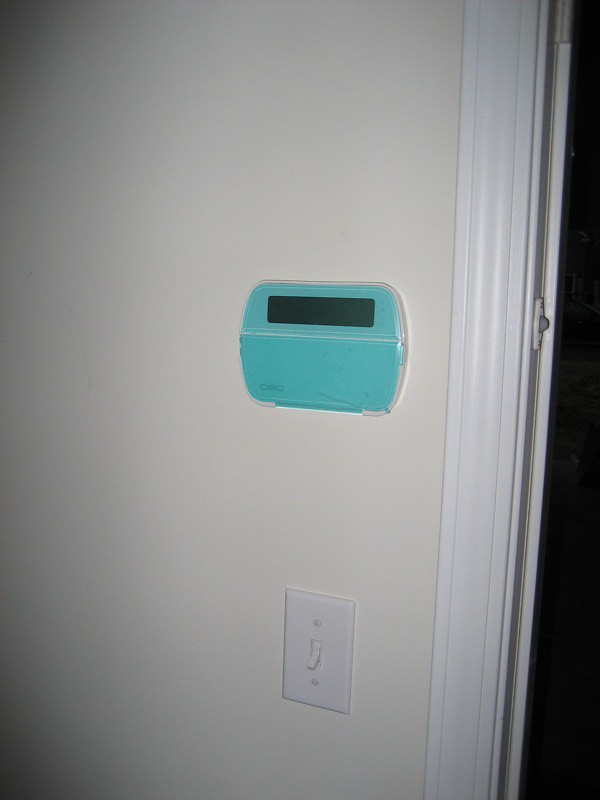In this image taken inside a house, we see an angled view of a white wall. On the right side of the wall, a white door is partially visible but not the main focus. Centrally featured on the wall is a small, teal-colored thermostat with an LED display bar that appears to be off. The thermostat has the text "OSC" written on its bottom left corner and is encased in a plastic covering. Below the thermostat, there's a single-switch switchboard with a protruding switch. The image also shows a vignette effect, with black shaded areas in the top left and bottom left corners.